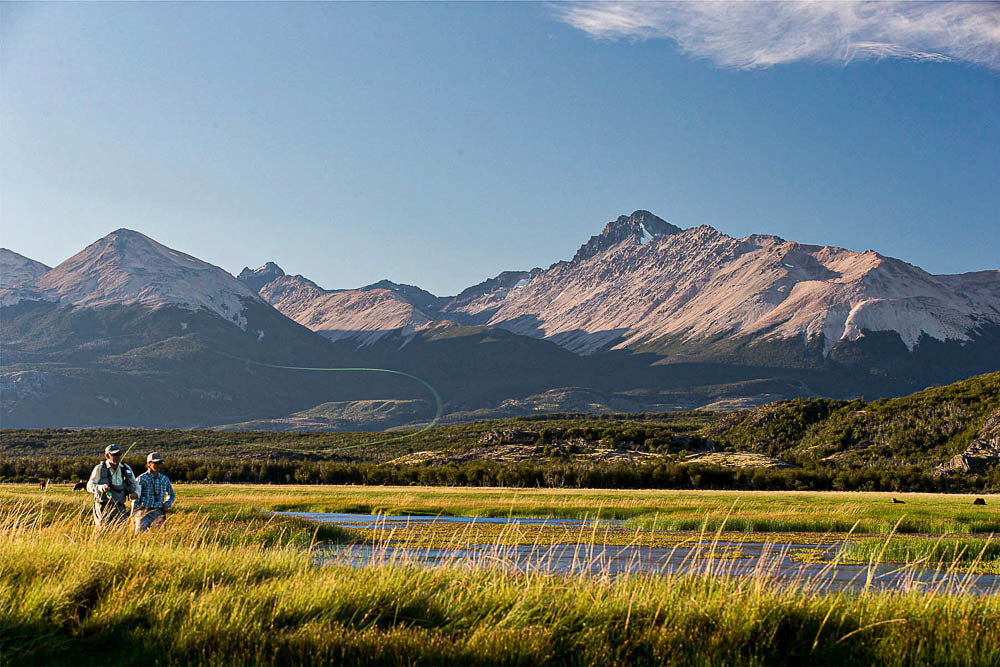In this captivating photograph taken during what appears to be either sunrise or sunset, a picturesque field stretches across the foreground. Dominating the scene is a bright green expanse where two men, dressed in fishing attire and hats, stand on the left side, seemingly preparing for a day of fly fishing. One of them is visible swinging a fishing pole, with the fishing wire caught mid-air. Just to their right, a serene pond occupies the center and right portion of the image, with a patch of green land situated in the pond’s midst. 

The bottom of the frame features tall grasses, green at the base and transitioning to tan at their tips, suggesting a lush yet wild terrain. Beyond this vibrant foreground, a small hill dotted with trees rises, leading the eye to the majestic mountain range in the background. The mountains showcase a picturesque display of various shapes and curves, many of which are snow-covered, providing a striking contrast to the greener lower slopes. 

At the very top, a light blue sky stretches across, decorated with just a singular cloud positioned on the top right, completing this serene and detailed natural scene.